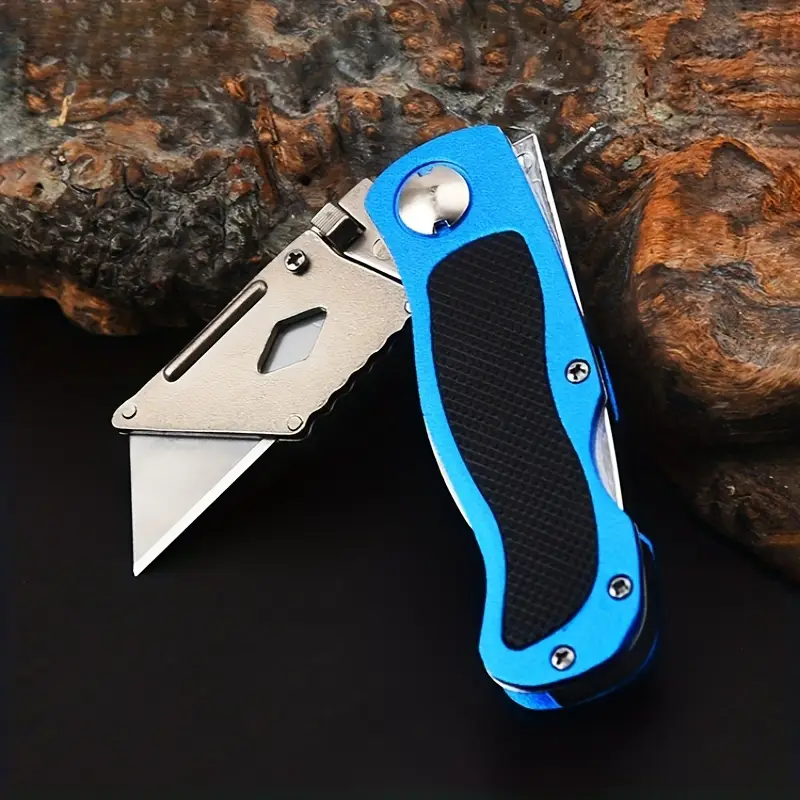This color photograph captures a detailed close-up of a multi-purpose knife, designed especially for utility cutting tasks. The knife, resembling a foldable box cutter, shines with a bright blue aluminum handle that is reinforced with a black rubber insert to enhance grip. The handle is meticulously held together by three Phillips head screws and a rivet, ensuring its rugged structure. Its replaceable, triangular razor blade is extended, ready for use. This versatile piece of equipment rests against a piece of gnarly, weathered wood, reminiscent of driftwood collected from a beach and stained a tan color, giving it a rustic, polished appearance. The overall composition is beautifully enhanced by the contrasting black surface beneath the wood, making the modern, robust design of the knife stand out vividly.